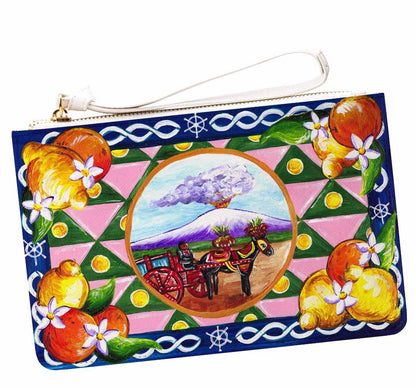The image depicts a small rectangular clutch purse, positioned slightly counterclockwise with a white handle attached to the zipper at the top. Dominating the center of the purse is a vivid circular illustration featuring a black donkey with an intricately designed saddle and cloth over its neck, pulling a red cart. The scene includes an erupting volcano with a cloud of ash in the background. This central image is bordered by an orange ring. Encircling this scene is a decorative pattern of green triangles set against a pink background, all encompassed by a blue border. Each corner of the purse showcases images of fruits and vegetables in shades of orange, yellow, and green, interspersed with white braid-like decorative elements, adding to the elaborate design.